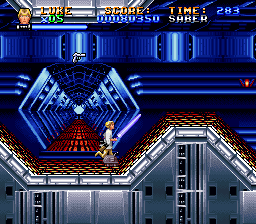A nostalgic screenshot from a retro video game, likely from the 80s or 90s, depicting a blonde man in a white shirt dashing through a futuristic environment that resembles a spaceship. The ground beneath him, vibrant with shades of orange and yellow, contours up and down, sitting atop a large metallic structure interlaced with additional metalwork. At the top of the screen, game stats are displayed: 'Luke' with a designation of 'X05', a score of '8350', a timer reading '283', and the term 'Saber' listed underneath the time. This classic vibe is emphasized by the pixelated graphics and simplistic interface, characteristic of that gaming era.